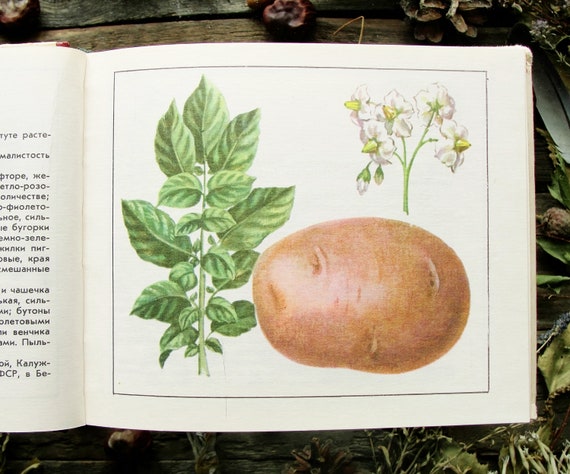The image depicts an open page of a book with a light yellow tint and a black border framing the illustration. Dominating the right-hand page is a detailed botanical drawing. On the left side of the illustration, a plant with a long green stem rises straight up, adorned with large, pointed leaves that vary in shades of green. Adjacent to this stem, at the bottom center, lies a large, light brown potato with several dents. Above the potato, a green stem emerges, splitting into three smaller stems that bear white flowers with yellow, pointed centers. The far left portion of the image shows a glimpse of the previous page, with some black text in an unrecognizable language. The book is laid out on a wooden table with plants, possibly potato plants, scattered around it. The setting, combined with the botanical focus of the illustration, suggests the page is from a detailed educational or scientific book about plants or vegetables.